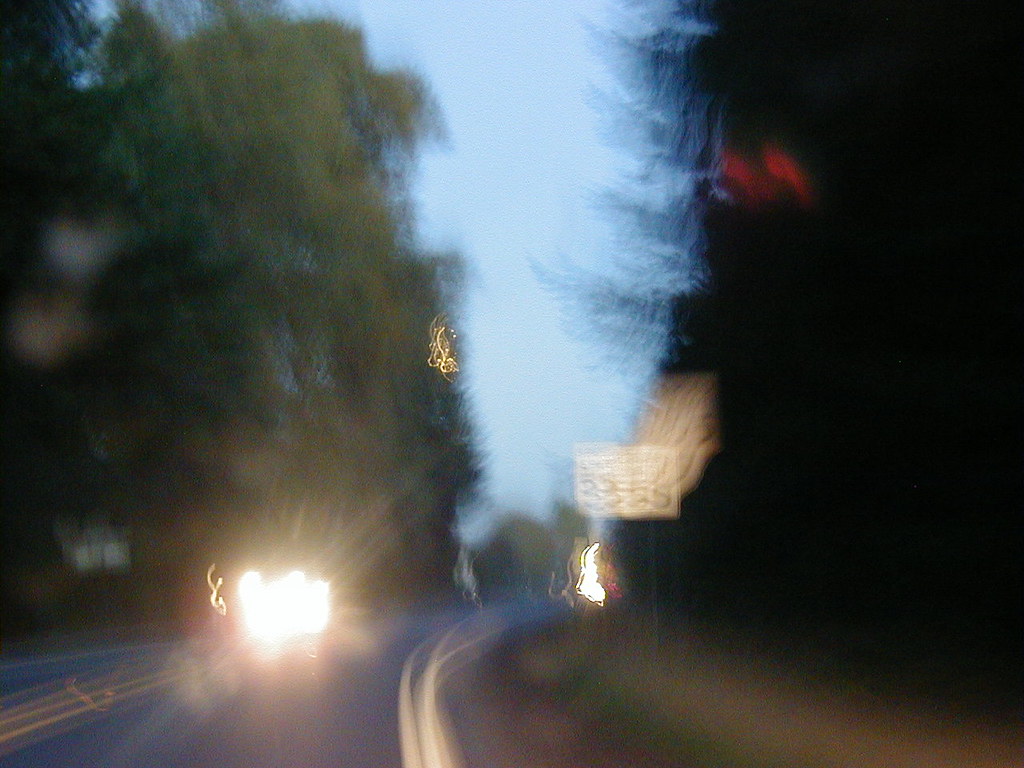This image captures a very blurred scene, likely photographed from a moving vehicle traveling down a highway. The driver is on the right side of the road, while another car is seen in the left lane, coming from the opposite direction. A clear no passing zone is indicated by two solid yellow lines down the center of the road. The lanes are marked with white lines, but there is no shoulder space visible on either side. A speed limit sign reads 35 mph, though it appears doubled due to the blurriness. Tall, densely packed trees line both sides of the highway, suggesting a heavily wooded area. The photo seems to have been taken either in the early morning or late evening, as the sun is not prominent, casting a dim light over the scenery.